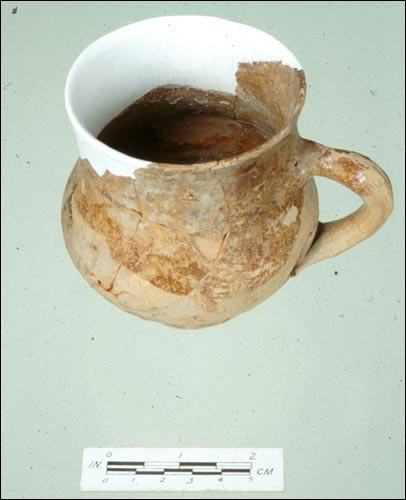The image depicts an ancient and unfinished clay drinking vessel, most likely a cup or a mug, identified by its medium to light brown hue and wide handle. The cup rests on a surface with a scale measuring in inches and centimeters, suggesting it is approximately three to four inches wide. The vessel's body features both rounded and unfinished clay sections, hinting it was partially painted white, while the rest retains the original clay texture. The mouth of the cup is as wide as its body, indicating a shapely and balanced design. The background of the image is a light bluish-green color, offering a pleasing contrast to the muted tones of the ancient cup.